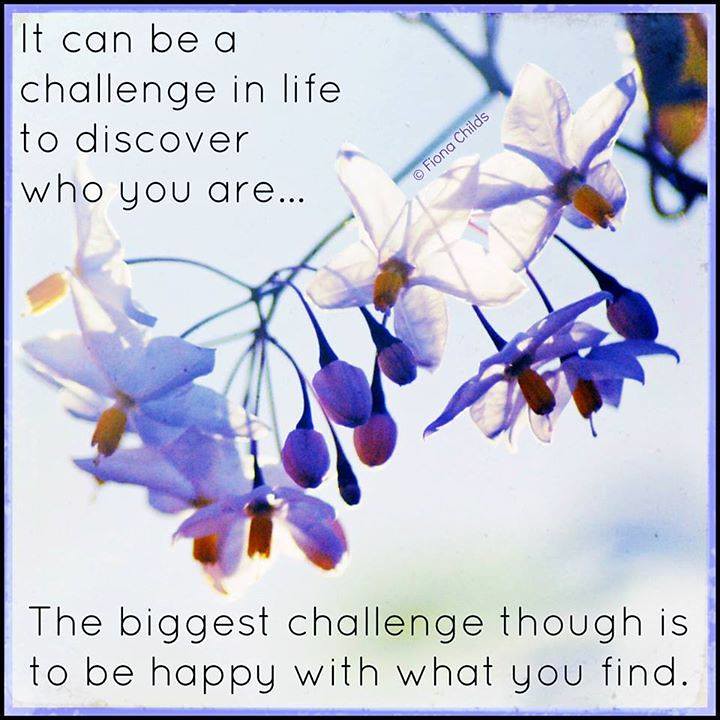This perfectly square, colored image features a close-up of a branch adorned with small white flowers, some fully bloomed with yellow centers while others remain as buds. The background is a bright, slightly out-of-focus sky, providing a serene backdrop to the delicate floral details. The image is framed with a black border, followed by a bluish-purple border. Text overlays the photo, with an inspirational message in black print: "It can be a challenge in life to discover who you are" positioned in the top left corner, and "The biggest challenge though is to be happy with what you find" stretching along the bottom. Above the flowers and the branch, there is a copyright notice that reads "Fiona Childs." This motivational image, with its blooming flowers symbolizing personal growth and acceptance, is well-suited for sharing on social media platforms like Facebook.